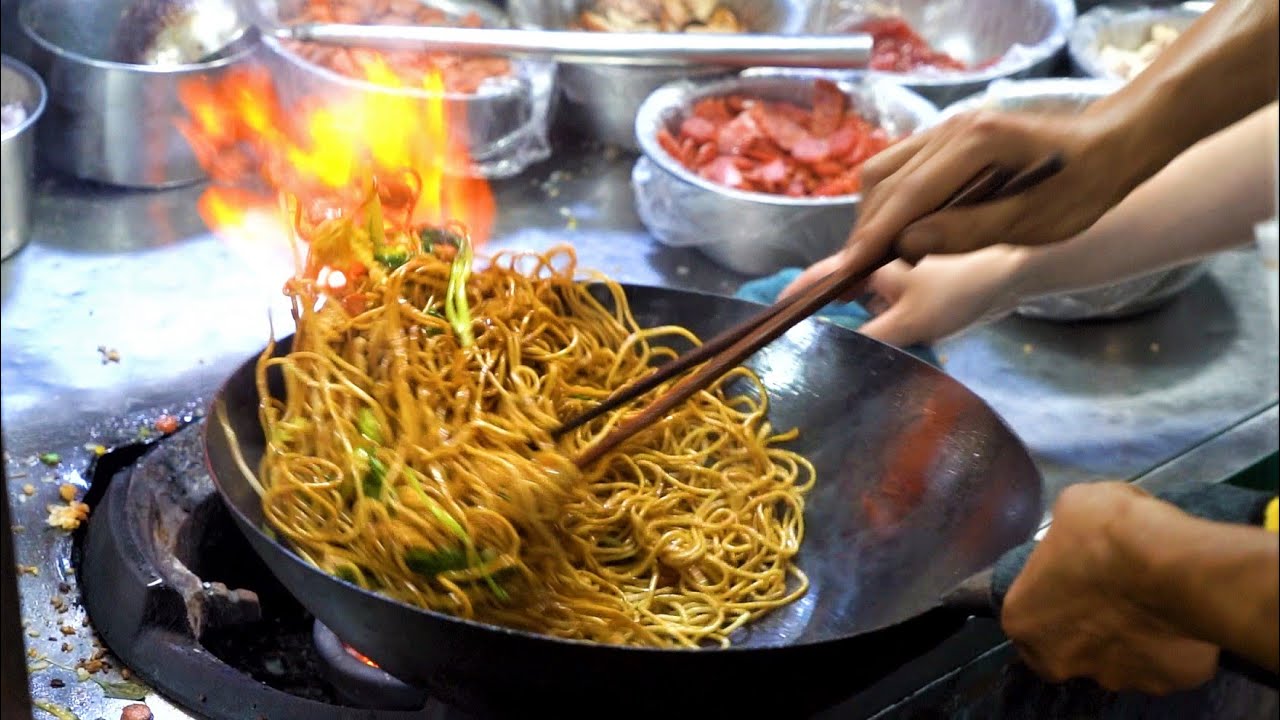This detailed photograph captures a dynamic cooking scene in a landscape orientation, possibly a freeze-frame from a video. At the heart of the image is a person with dark skin, skillfully preparing a stir-fry dish, most likely chow mein, using a round, large cast-iron wok with a metallic black finish. The wok features a handle, which the cook grips with a black towel in their left hand. Meanwhile, their right hand masterfully maneuvers long brown wooden chopsticks to stir the sizzling noodles and green broccoli.

The vigorous cooking process is accentuated by flames that dance and flicker up behind the wok, illuminating the stir-fry. The wok itself is centered in a recessed cooking area with an open flame, integrated into a stainless steel cooking surface. Surrounding the central action, multiple bowls containing various chopped and prepared ingredients are arranged, ready to be added to the meal. A large metal ladle rests in a pot filled with sauce, also visible among the array of cooking tools. The photograph encapsulates the intense, vibrant moment of cooking, blending the heat of the stove with the rich colors and textures of the ingredients.